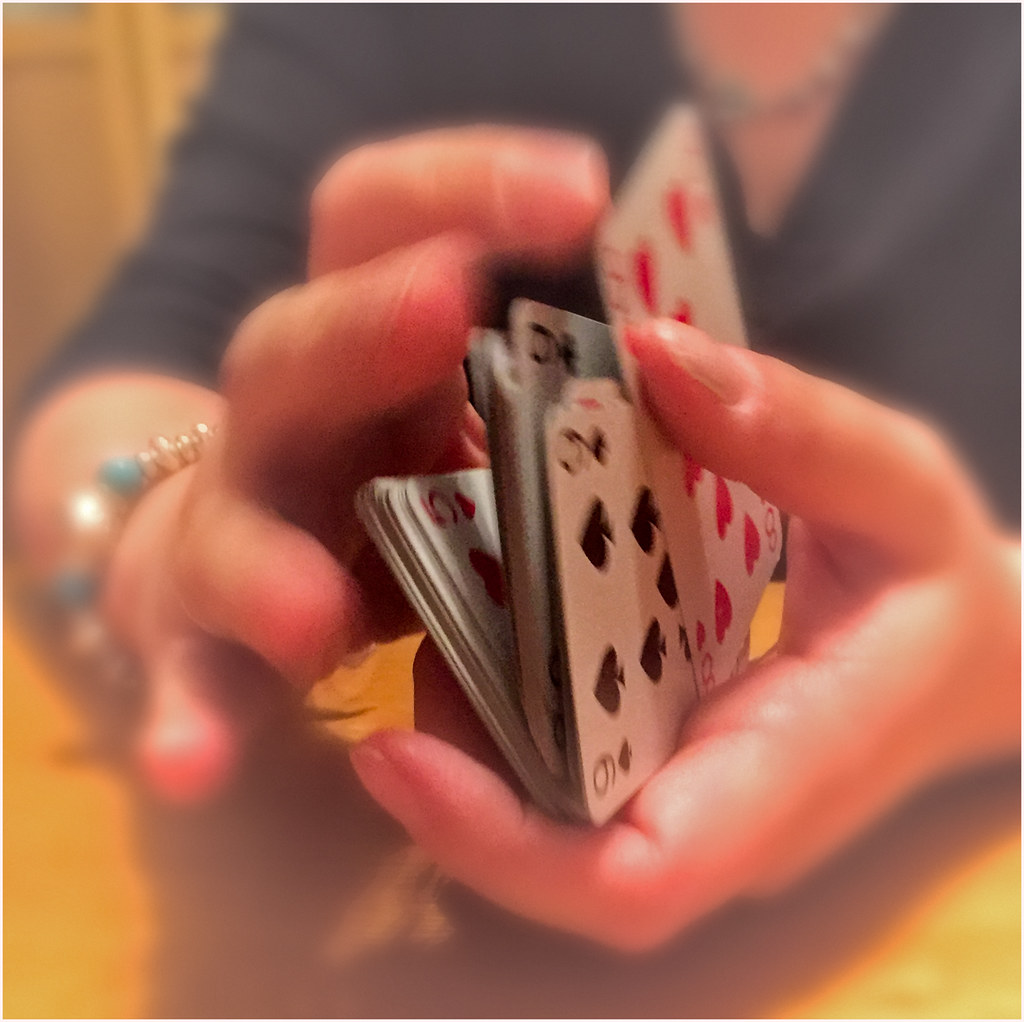In the image, a pair of hands is caught in the act of shuffling a deck of cards. The hands, whose gender is indeterminate, sport a bracelet on the right wrist, positioned on the left side from our perspective. The bracelet features an array of beads: four small silver ones interspersed with larger beads in a pattern of blue, white, blue, white, and blue. The person's sleeves are rolled up past their elbows, exposing the majority of their forearms, and they are dressed in a V-neck shirt with a necklace faintly visible beneath it. The scene is set against a yellow table, with yellow wooden elements in the background. Shadows of the hands dance across the surface. Among the deck, a few cards are distinguishable - a nine of spades, a five of hearts, and possibly another nine of clubs. Another five of hearts is seen further back in the shuffled deck.